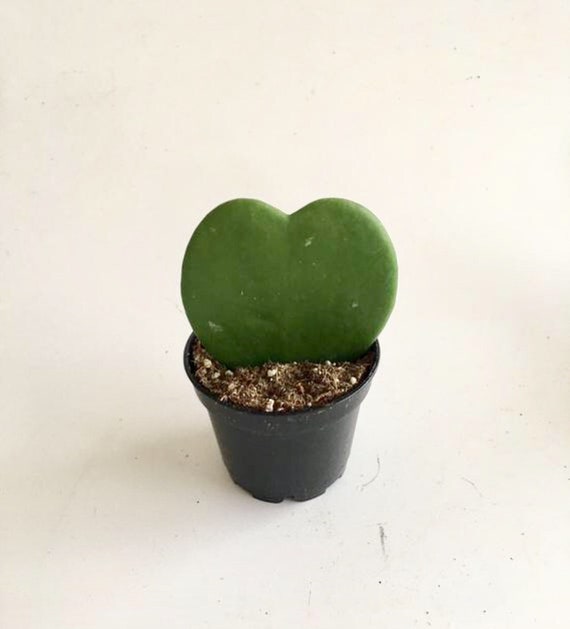This photo depicts a small, dark-colored flower pot, almost black or very dark brown, which is simple and unadorned. The pot is filled with brown soil sprinkled with white specks, and appears somewhat bucket-shaped. Inside, there's a single green plant that strongly resembles a cactus but without any spines. The plant is a vibrant green, shaped distinctly like a heart or a filled-in, rounded letter M. Its form is smooth, lacking any leaves, and has occasional white flecks on it. The entire scene is set against a plain, pale background, ranging in description from beige to light gray, with no visible lighting or shadows, giving the image a very clean and minimalistic appearance. Additionally, the photo itself seems to have some dirt marks or blemishes.